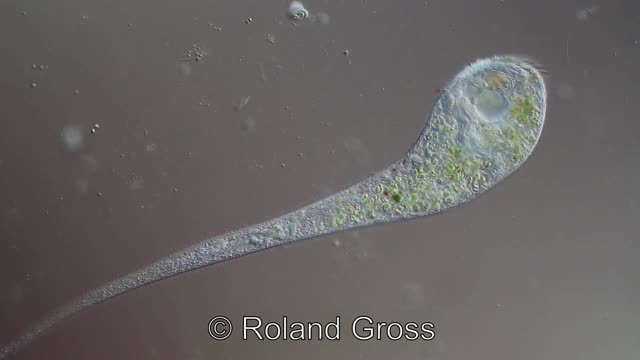This photograph, credited to Roland Gross, displays an organism under a microscope with a predominantly gray background, interspersed with a few white circles and cylinder-shaped objects. The organism, which appears to be a form of bacteria, has a long, worm-like body that starts off thin at one end and progressively widens, tapering into an oval shape towards the middle before extending into a long tail. The central oval region of the organism is characterized by a divot, possibly an eye, which is larger and flatter. The organism exhibits a bluish-gray coloration with mold-like, green specks scattered across its surface, giving it a bumpy texture. The bottom of the photo prominently features the copyright notice for Roland Gross in white letters.